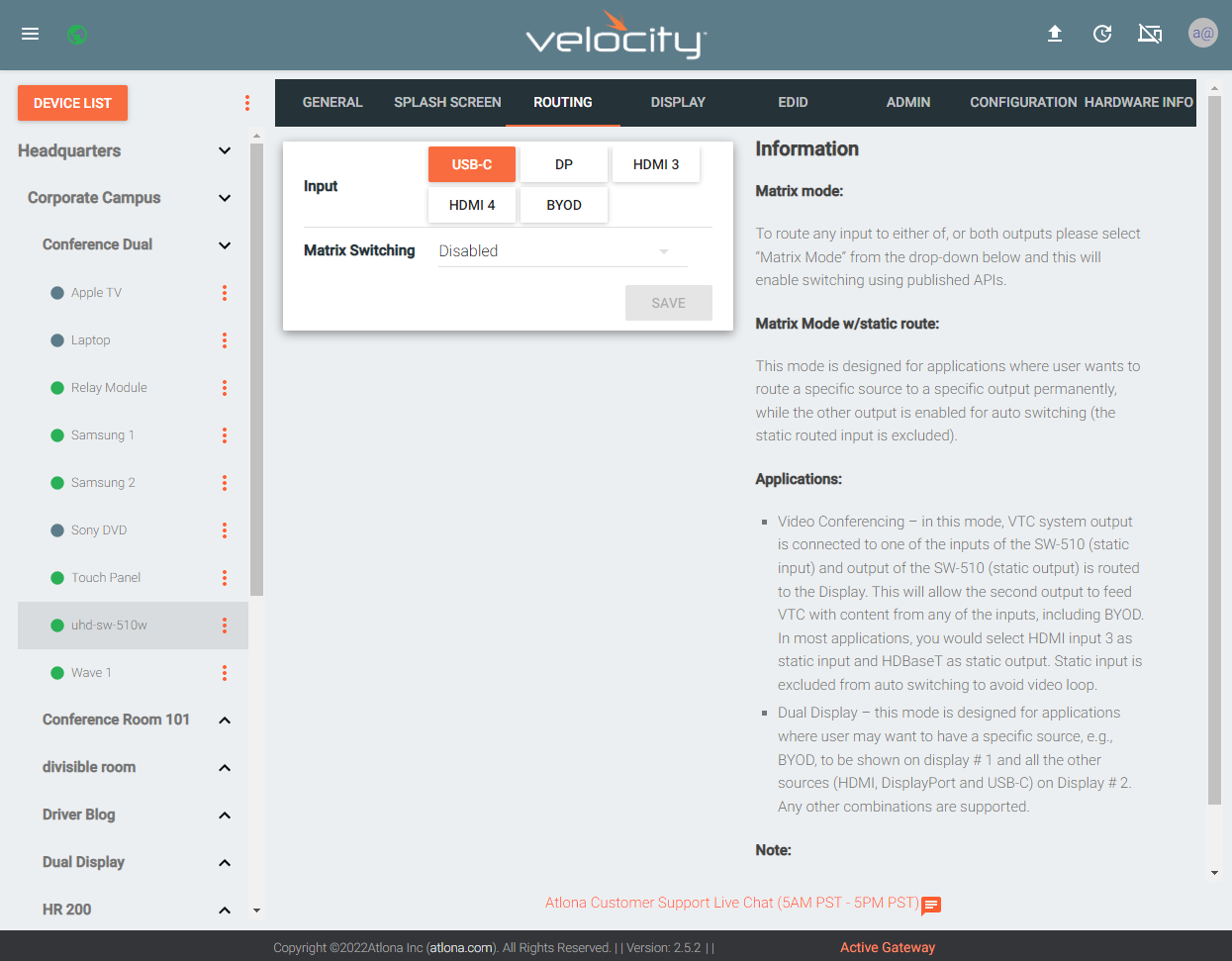The screenshot features the interface of the app "Velocity." In the center of the screen, the word "Velocity" is displayed in white lettering, accompanied by an orange plane-like icon pointing towards the 'C'. 

The top navigation bar lists several categories: General, Splash Screen, Routing, Display, EDID, Admin, Configuration, and Hardware Info. The current selection is "Routing." 

In the main section, the interface displays several input options, with USB-C highlighted in orange, indicating it is currently selected. The other input options include DP, HDMI 3, HDMI 4, and BYOD, none of which are highlighted. 

Below, there is a category for Matrix Switching, which is set to "Disabled." The Save button is grayed out, likely requiring a change in settings to be activated. 

Information about Matrix Mode is provided: 
- To route any input to either or both outputs, Matrix Mode must be selected from a drop-down menu.
- Enabling Matrix Mode facilitates switching using published APIs.
- The Static Route mode is designed for applications that require a specific source to be routed to a specific output permanently. Even when the output is enabled for auto-switching, the static route input remains excluded. Applications for such settings include Video Conferencing and Dual Display.

On the left side, there are drop-down categories such as Headquarters, Corporate Campus, and Conference Dual. Under these, controllable devices are listed, including Apple TV, Laptop, Relay Module, Samsung One, Samsung Two, Sony DVD, and Touch Panel. Currently, the UHD-SW510W Wave 1 device is selected. 

Further down, additional categories such as Conference Room 101, Divisible Room, Driver Blog, Dual Display, and HR-200 are listed, presumably for specific control settings. 

The interface appears to offer comprehensive control over various devices and room settings within an organizational infrastructure.